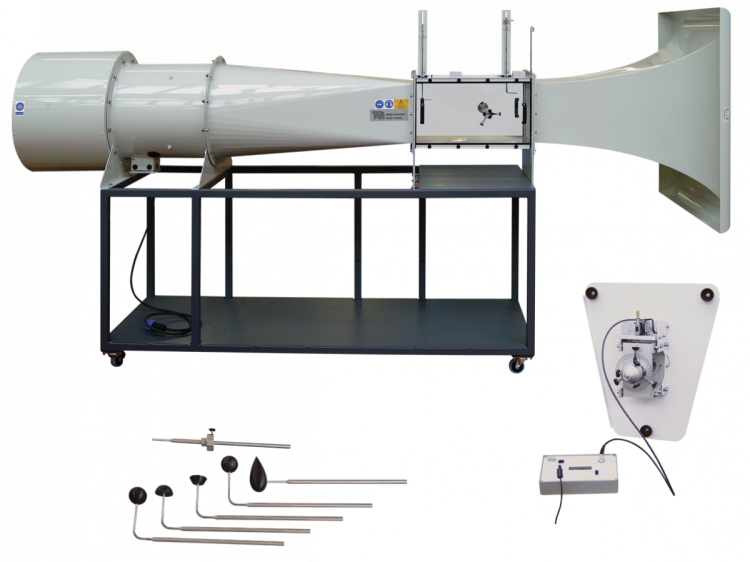The image depicts a large, metallic off-white cylindrical scientific instrument mounted on a black trolley with wheels. The right end of the cylinder transitions into a rectangular cone that resembles a wind tunnel, and there's a clear box-like section in the middle. Electrical cords are seen hanging from the instrument. Below the main device, there are several smaller metallic instruments of various shapes and sizes, including components with circles on the ends, some resembling hammer-like tools, and a probe. On the bottom left, there is another piece of equipment that appears to be a white switch with wires. On the bottom right, an instrument with a gauge and monitor, potentially a part intended to attach to the main cylinder, is visible. The overall setup appears quite modern, though the specific purpose of this equipment is unclear.